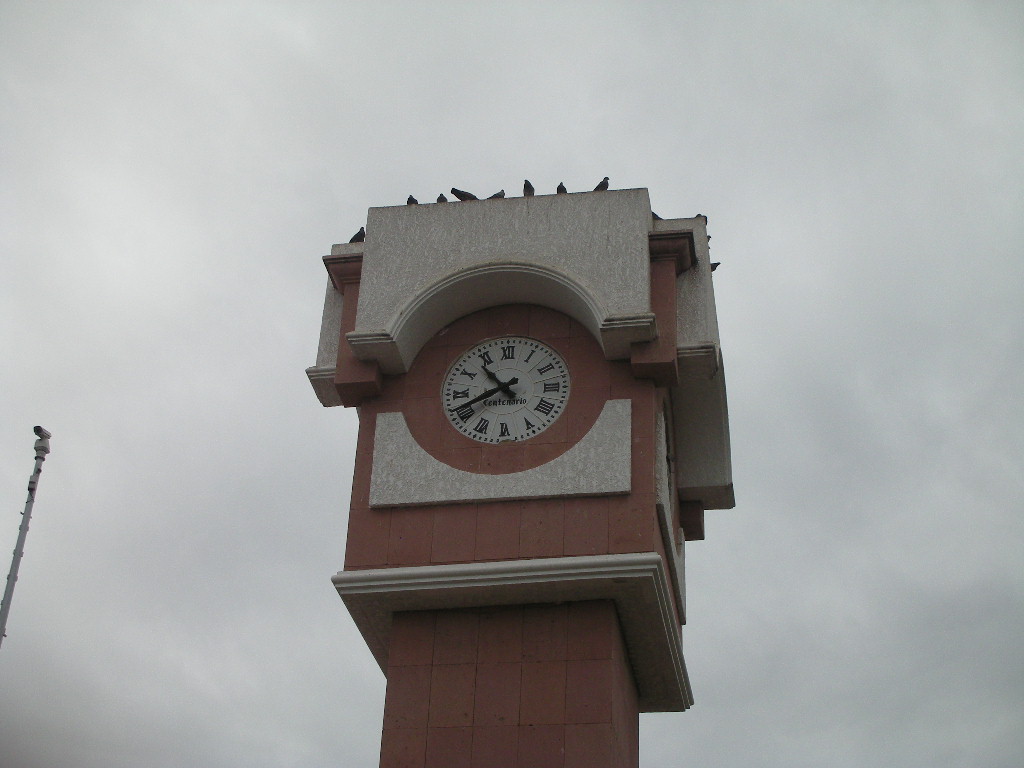A towering clock stands majestically on a red brick pedestal, its impressive height emphasized by the upward camera angle. The clock features a round face enclosed in a gray stone-like frame, an elegant contrast to the rich red bricks beneath. Black hands—one short, indicating the hour, and one long, representing the minutes—gracefully tick along the clock's surface, which stylishly displays Roman numerals instead of traditional numbers. Perched serenely at the peak of this monumental structure are numerous birds, adding a touch of life to the scene. The photograph captures not only the intricate details of the clock but also its commanding presence in the environment.